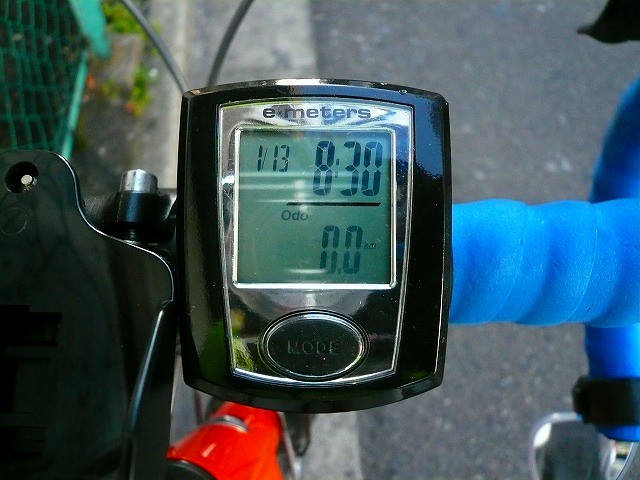In this outdoor photo, a bicycle is prominently featured on a dark street, with a lighter gray curb visible in the background. A green fence lines the backdrop, adding to the scene's vivid detail. The bicycle is equipped with an "E-Meters" tracking device, a black rectangular component that displays the numbers "1-13-8-30" and indicates no recorded distance traveled yet. Below these numbers, there's additional text that is unclear, possibly reading "R-O-P-E" or "K-O-P-E." An enigmatic orange object, potentially a cone, is also visible in the background. The bicycle's blue handle transitions into a gray metal or chrome section. On the left side of the bike, something black appears to be attached with screws or nails, which may be a holder for a phone or another accessory.